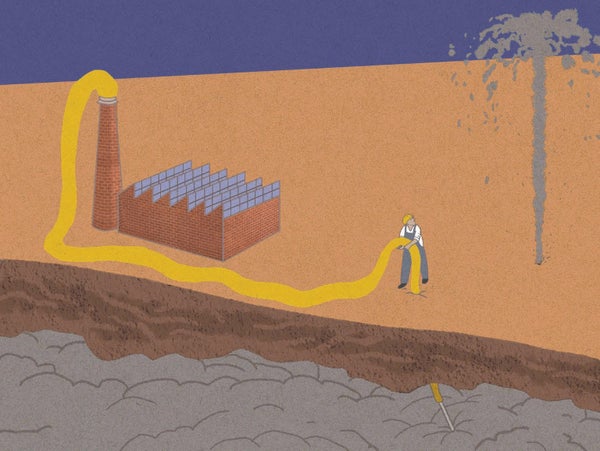This detailed illustration depicts a man dressed in blue overalls, a short-sleeved white t-shirt, black boots, and a yellow hard hat. He is holding a large, gold-colored hose that extends from a brick smokestack on the right side of the image. The hose penetrates the earth's surface, which is a tan color, and burrows through the first layer of brown soil into a darker gray layer, presumably filled with oil. To the right of the man, an oil geyser is visibly erupting from the ground. Further to the right, a series of solar panels are shown lined up. The scene offers a cross-sectional view of the earth's layers with a clear representation of the ground and subsurface layers. The man appears focused on the processes occurring around him, particularly the oil gushing up, which contrasts sharply with the orderly row of solar panels leading to the industrial smokestack.